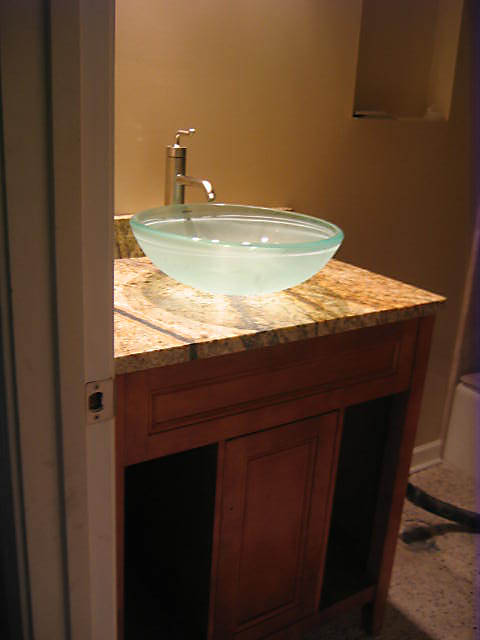In this indoor color photograph taken under dim lighting conditions, the viewer's perspective is through a doorway leading into a bathroom. Dominating the left side of the image, a door jamb stretches vertically from the bottom to the top edge, featuring a visible striker plate in the center. The focal point of the image is a luxurious dark brown marble countertop centrally situated, boasting subtle light tan veining. 

Atop the countertop rests a sizable frosted glass basin, approximately 20 to 25 inches in diameter. Directly behind the basin stands a sleek, polished stainless steel faucet. The faucet's cylindrical base rises vertically before extending a spigot out horizontally at a precise 90-degree angle, which then bends downward at a 45-degree inclination into the bowl. At the spigot’s apex is a solitary control lever.

Beneath the countertop, the bathroom vanity showcases rich, dark wood paneling, adding depth and contrast to the scene. The background wall is painted a soft light tan, providing a neutral backdrop. In the photograph's lower right corner, part of the floor is barely visible, potentially comprised of light tile, though the details are indistinct. 

An unadorned rectangular mirror, possibly part of a medicine cabinet, occupies the upper right corner, reflecting the tan wall behind it. The overall photograph is slightly out of focus and enveloped in dim light, lending a soft and subdued ambiance to the space. No text, words, or prints are present within the frame.